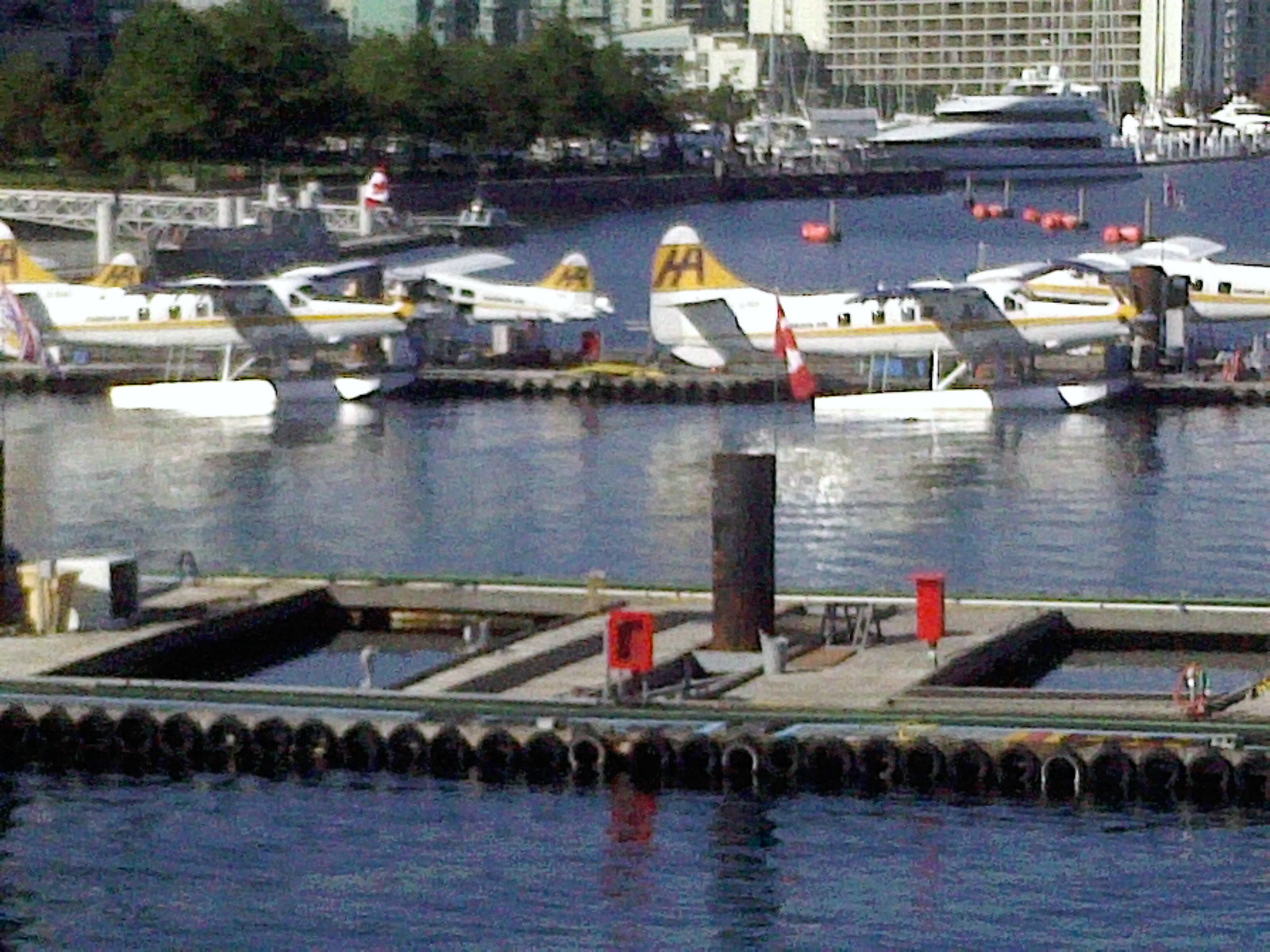The image captures a bustling harbor scene on a calm, sunny day, characterized by its grainy, low-resolution quality indicative of an older photograph. In the foreground, an empty dock leads to a floating dock in the midground, where two white float planes with yellow striping and "HA" on their tails are moored. These planes are equipped with prominent white floats attached to their legs. To the top right, a large, multi-level white yacht is anchored, positioned near a building with numerous balconies, which could be a hotel or office complex. Further into the background on the left, a line of green trees borders the port, while in the top far right, the building bears resemblance to a parking garage. Red buoys dot the water near the yacht. The harbor's water is calm, with only small ripples, reflecting the float planes and docks clearly. The bright and sunny conditions enhance the overall scenery, casting a lively ambience over the port.